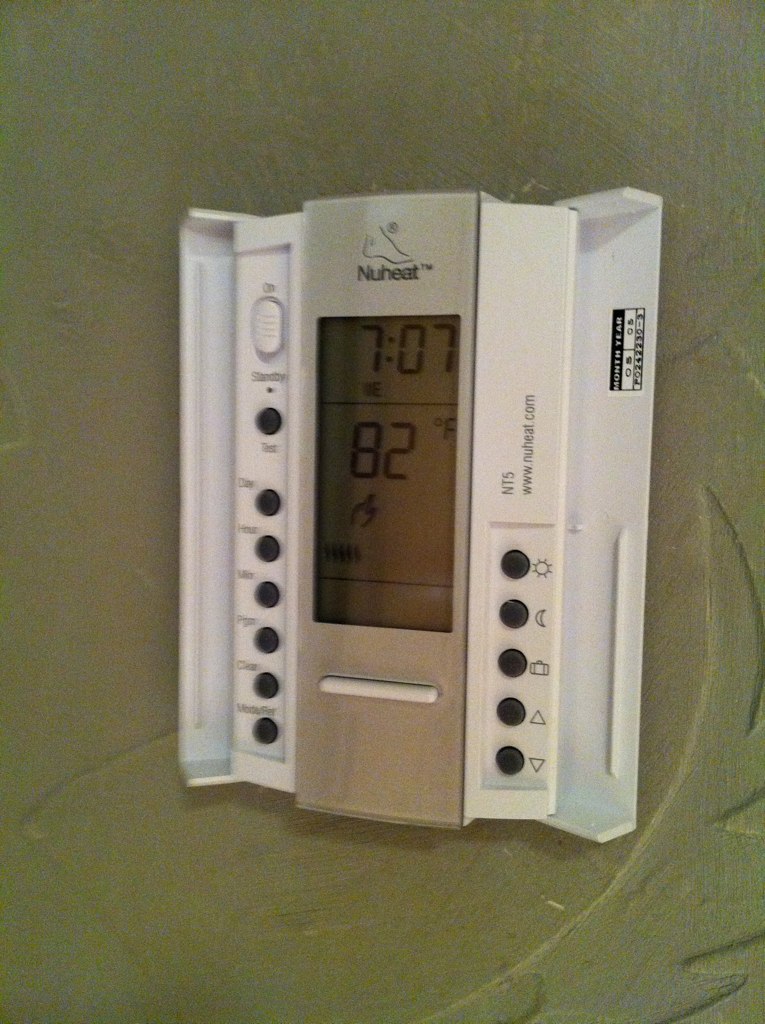Mounted vertically on a tannish-brown wall with a subtle leafy design, this thermostat, branded "New Heat" in black lettering, features a unique and intricate setup. The thermostat's cover, which opens like a book or a box top on both sides, reveals an array of controls and a digital display. 
At precisely 7:07 (the time being indiscernible as AM or PM), the digital screen prominently shows a temperature of 82 degrees Fahrenheit. On the left side of the device, there are seven black buttons arranged in a vertical row, topped by a distinct oval white button, likely serving as the power button.
The right side presents five black buttons, with the bottom two featuring triangles pointing downward and upward, presumably for adjusting the temperature. Additional black buttons have unspecified functions. The inner lid on the right side has a vertical black rectangle containing some text, which is unclear in detail.